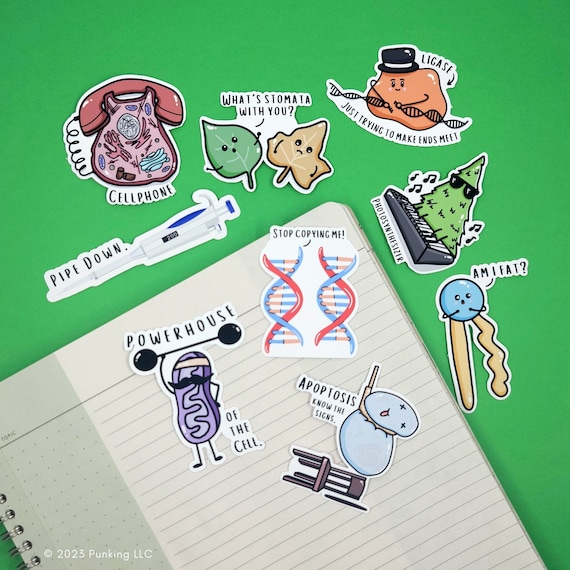The image features a collage of computer-animated stickers on a green background, resembling a piece of notepad paper. On the top left, there's an old-fashioned pink rotary phone labeled "cell phone." To the right, a pair of leaves, one green and one brown, are depicted with faces, accompanied by the text "What's the matter with you?" Further to the right, a potato with a small black hat and a smiling face is labeled "Just trying to make ends meet." Below the potato, a peanut character with arms, legs, and a mustache is seen lifting a large weight, with the caption "Powerhouse." Additional elements include a piano-playing tree labeled "photos you synthesizer" and a light blue character with X's for eyes labeled "apoptosis know the signs."